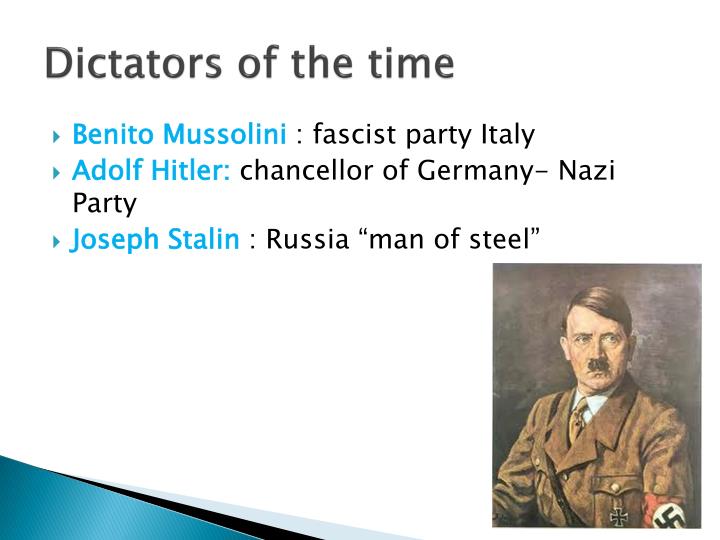The PowerPoint slide features a white background with a slight design element in the bottom left corner, comprising a blue triangle with black and gray slashes. The main title at the top reads "Dictators of the Time" in a black font. Below this, three bullet points provide details about key dictators. The first point reads "Benito Mussolini: Fascist Party, Italy," with the name in light blue text. The second point is "Adolf Hitler: Chancellor of Germany, Nazi Party," also in light blue text, whereas the rest of the text is in black. The third point states "Joseph Stalin: Russia, 'Man of Steel,'" with the name in blue and the rest of the text in black. On the bottom right side, there is a portrait of Adolf Hitler, showing him looking serious with slicked-back brown hair, a center mustache, a brown jacket, a white shirt, and a yellow tie. He is wearing a red armband with a black swastika in the middle. This detailed slide effectively captures information about these notorious historical figures.